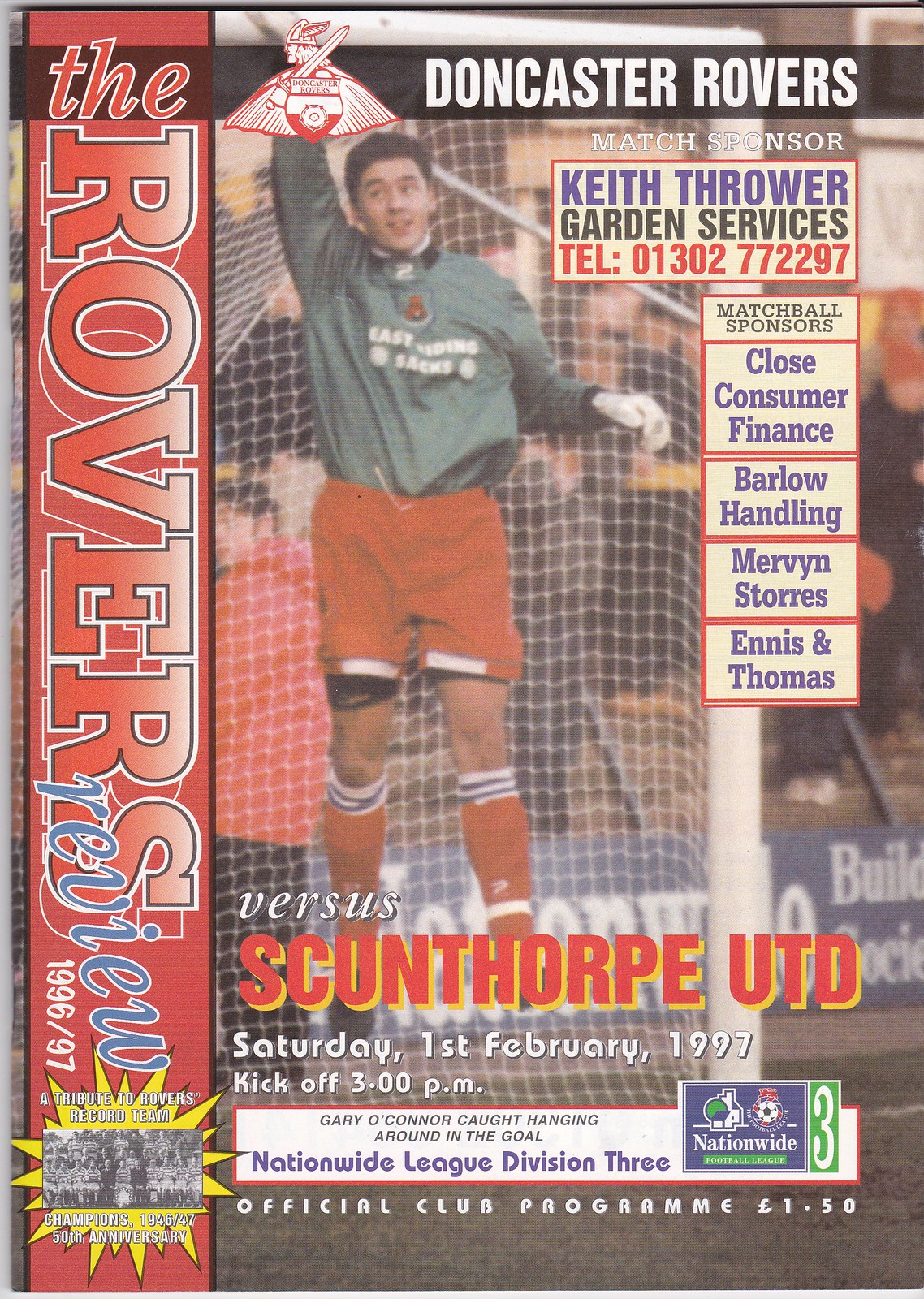The cover of the magazine features a striking layout with a red vertical strip on the left side, which is inscribed with the magazine's title, "The Rovers Review 1996-1997," vertically in blue letters. Adjacent to this strip, a dynamic image of the team's wicketkeeper stands out. He is clad in a dark green long-sleeve shirt, red shorts, and red knee-high socks, positioned in front of a net. At the top right corner of the cover, a horizontal black band boldly displays the text "Doncaster Rovers" in white. Below this, there’s further information about match sponsors, including "Keith Thrower Garden Services" with a contact number, followed by additional sponsors: Close Consumer Finance, Barlow Handling, Merlin, Mervin Store, Ennis, and Thomas. Towards the bottom center of the cover, detailed text outlines the upcoming match details: "Versus Scunthorpe UTD, Saturday 1st February 1997, Kick-off 3.00pm." Moreover, it is noted that this is the official club program, priced at one and a half pounds.